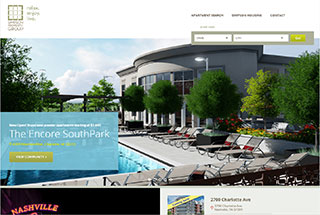In this screenshot of a website, the image appears small and pixelated. The logo, located in the upper left corner, is a green square with grid lines dividing it into nine smaller squares. In the upper right corner, there are three clickable tab buttons, positioned above two dropdown menus. The dropdown menu on the left is smaller than the one on the right. To the right of these dropdown menus is a green button. 

Further down, the main section of the image displays a photograph of a public pool area surrounded by chairs and trees. Superimposed over the photo is a rectangular text box that reads "The Encore South Park," with another green button positioned beneath it. 

At the bottom of the screenshot, the lower left corner shows a cropped image of a sock with the word "Nashville" from another photo. Meanwhile, in the lower right corner, there's an address accompanied by a photo that resembles the exterior of a hotel.